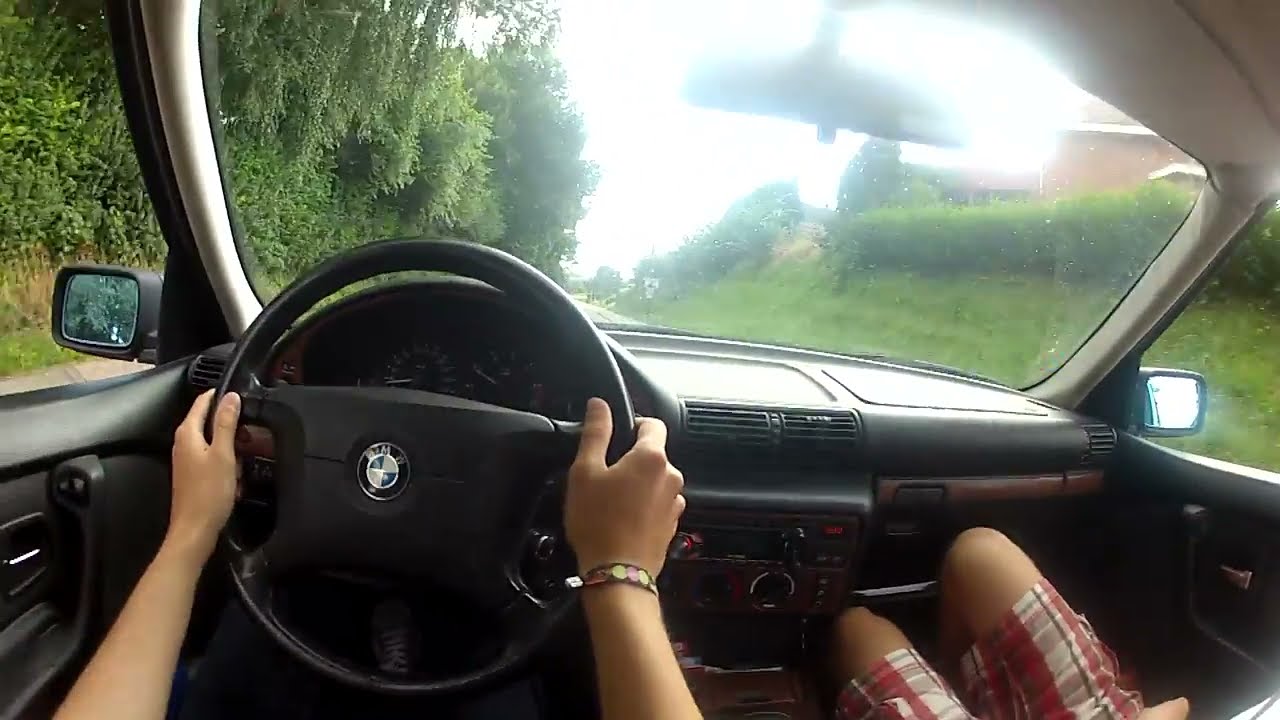This is an image captured from the perspective of the driver inside a BMW with a grey interior accented with beige on some posts and the roof. The driver’s forearms, adorned with a brown bracelet featuring yellow and pink circles on the right wrist, are firmly placed on a black steering wheel bearing the BMW logo in its center. The view through the windshield reveals a tree-lined road under a bright sky, with a brick house on the right side. In the passenger seat, a small child wearing red, white, and black plaid shorts sits uncomfortably, their knees pressed against the glove box. The car windows and mirrors frame the vibrant outdoor scene, with tall trees and bushes visible on either side of the car.